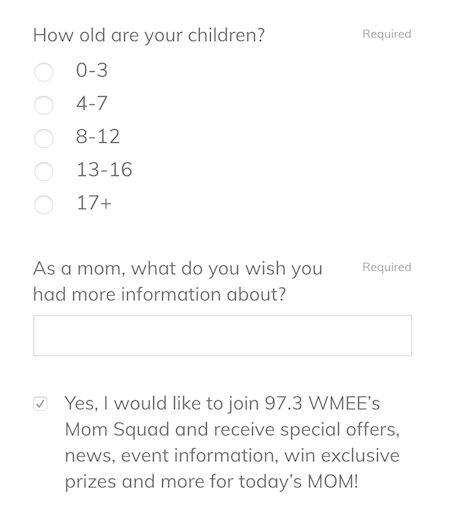The image depicts an online sign-up form for 97.3 WMEE's "Mom Squad," presented on a clean, white background with predominantly gray and black text. The form is designed to gather specific information from users, starting with a required question: "How old are your children?" The available options are presented with small circles to the left, each indicating an age range: 0 to 3, 4 to 7, 8 to 12, 13 to 16, and 17 plus. The subsequent prompt asks, "As a mom, what do you wish you had more information about?" This field is also mandatory but currently blank in the image. At the bottom of the form, there is a checkbox allowing users to opt-in to join the "97.3 WMEE Mom Squad," which promises access to special offers, news, event information, exclusive prizes, and other benefits tailored for modern moms. The overall aesthetic is straightforward and user-friendly, with a primary emphasis on ease of readability and clarity. The impression suggests that this form is part of an initiative from an out-of-state radio station, 97.3 WMEE, to engage and support its listener base, particularly moms.